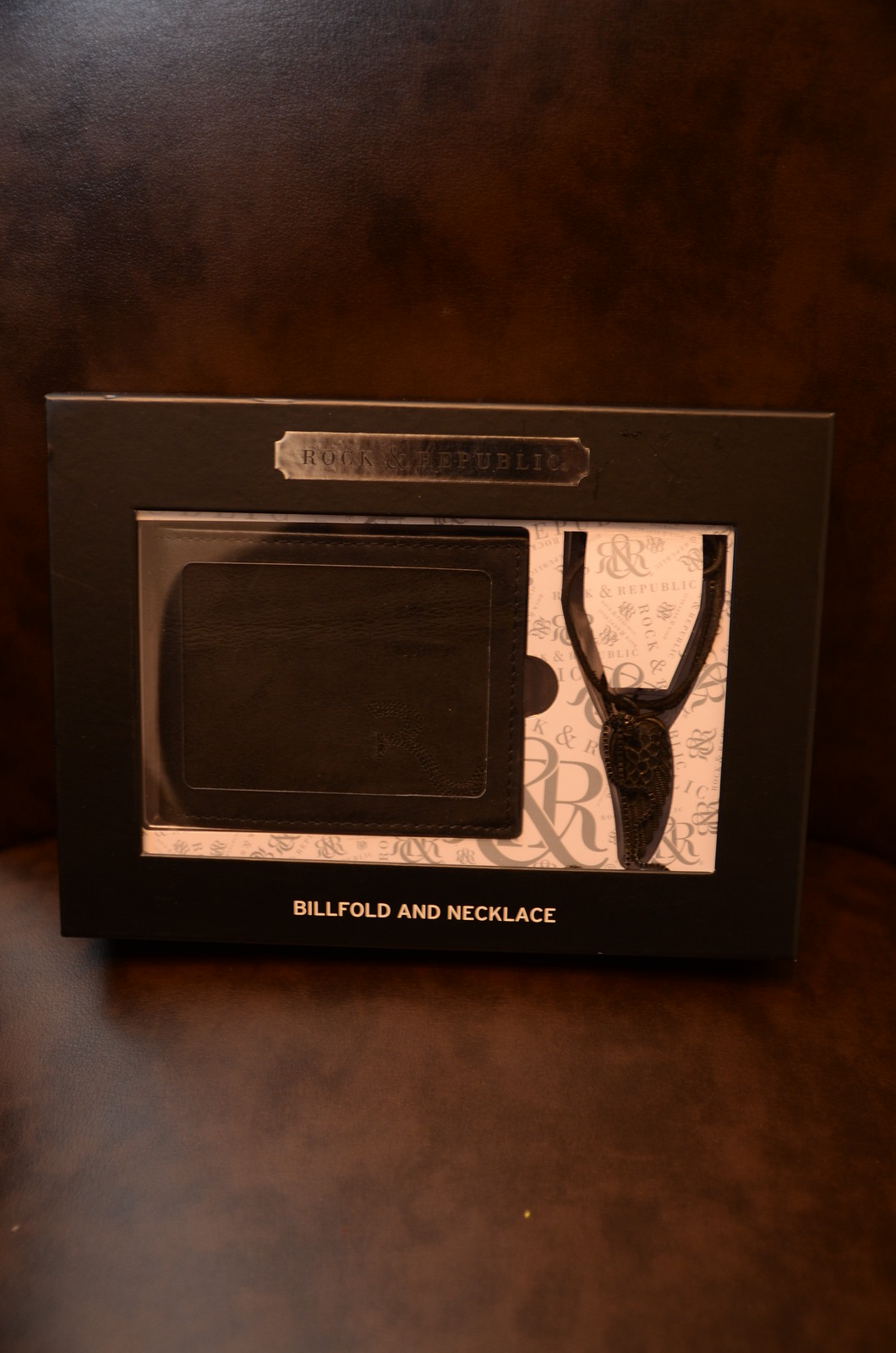The image is a black-and-white photograph featuring a boxed set that includes a billfold and a necklace. The box has a transparent cover, allowing a clear view of its contents: a brown leather wallet on the left and a necklace with a wing-shaped pendant on the right. A nameplate at the top of the box, partially legible, seems to say something like "Rock Republic." In white letters at the bottom of the box, it clearly reads "billfold and necklace." The background of the image mimics a brown, marbleized or leather texture, and the lighting is brighter in the top left corner, casting a gentle glare on the bottom left.